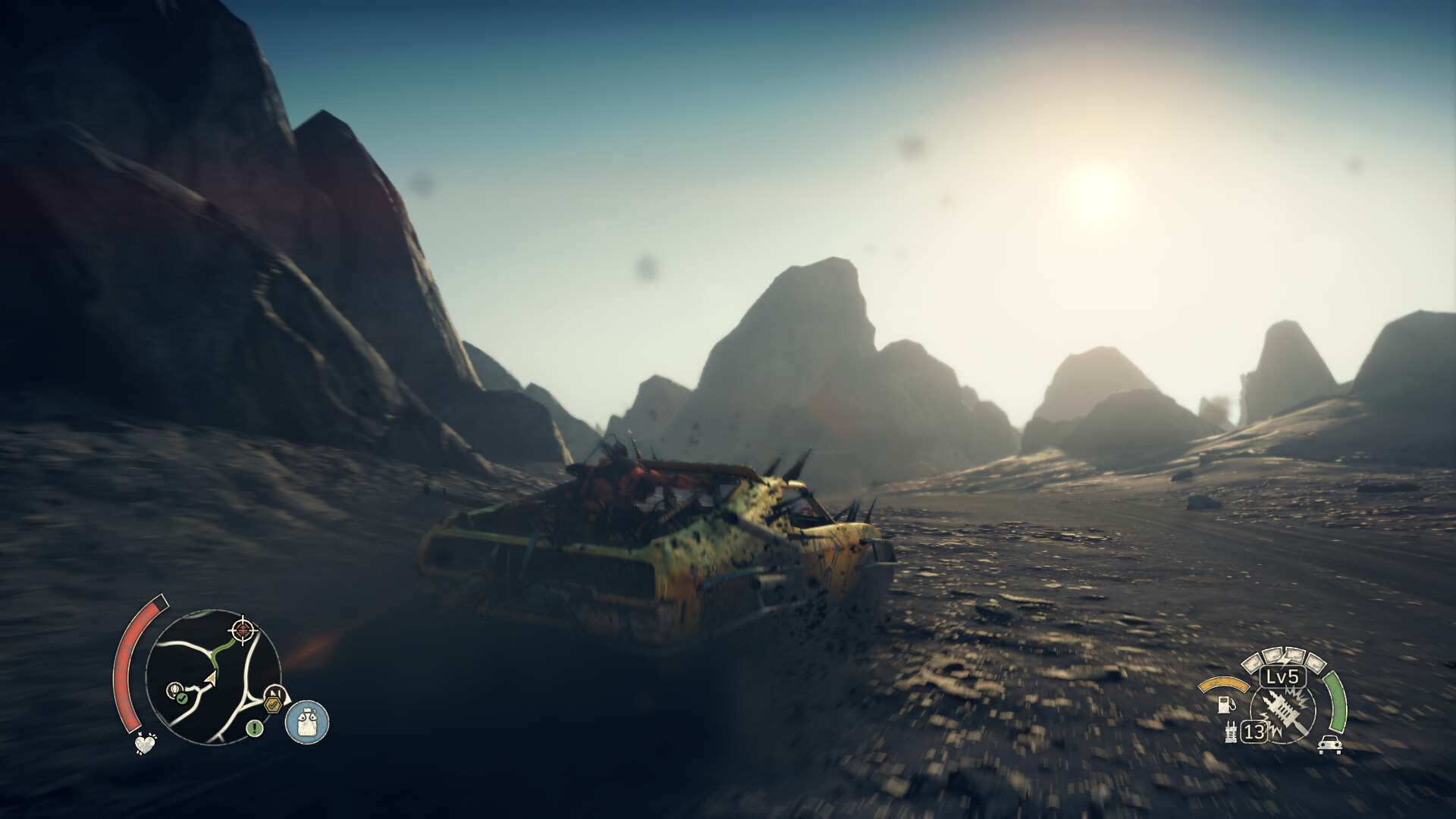The image appears to be a screenshot from a post-apocalyptic video game, capturing a barren, desert landscape under a clear sky with the sun low on the horizon. The terrain is rugged and mountainous, devoid of any vegetation. In the foreground, a battered, yellowish vehicle resembling a hybrid between an 80s El Camino and a pickup truck drives across the desolate scene. The vehicle is heavily modified, adorned with spikes and potential weaponry, suggesting a need for defense or combat.

In the bottom left corner of the screen, a mini-map is visible, featuring a curved bar that is predominantly red with a hint of black at the end—possibly indicating health status or proximity to a goal. The bottom right corner displays additional heads-up information, including an icon of a fuel tank that is entirely filled, and indicators showing "Level 5" and the number "13." There is also a green curved bar with an icon of a car, likely signifying the vehicle's current undamaged condition.